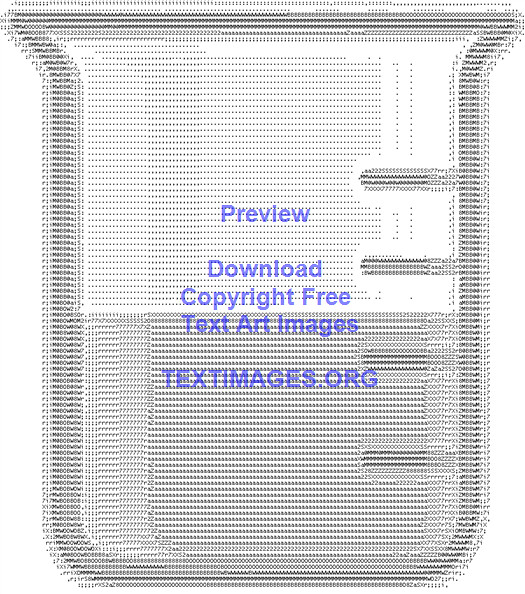The computer-generated image features a white background with a floating design, where numerous small dots and text characters form the shape of a science lab beaker. This beaker-like figure, without any outline, utilizes various shades of gray and white to define its structure. On the right side of the beaker, there are four measurement marks ascending vertically. At the center of the beaker, bold purple text reads "Preview," followed by "Download Copyright-Free Text Art Images." Below this, the website "textimages.org" is displayed, suggesting a place to access and download similar text-based art images. The overall appearance resembles an advertisement for text art imagery.